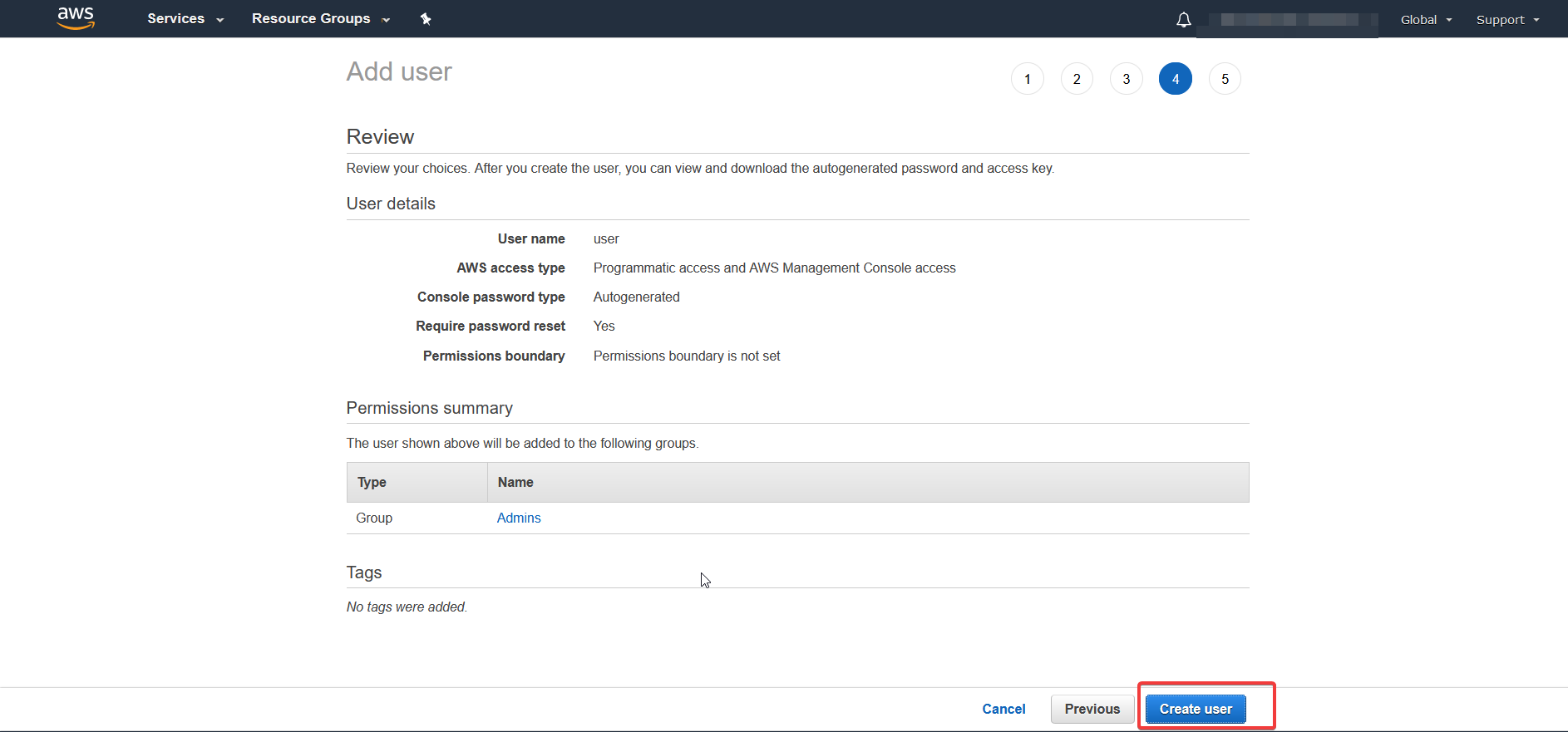The image displays a user interface, specifically likely from an AWS (Amazon Web Services) management console. At the top, a black bar contains the AWS logo alongside a symbol, and the words "Services" and "Research Groups" in dark blue or black text. A bell icon and additional text are present but not legible. 

Below the black bar, in gray text, it says "Add User." To the right of this, the numbers 1, 2, 3, 4, and 5 are displayed horizontally, with the number 4 encircled in blue, indicating the current step. In bold text, the word "Review" is shown, followed by "Review your choice."

Further down, a section titled "User Details" appears. In bold, it states "User Name" next to the label "User AWS Service Type". The text becomes increasingly difficult to read here but mentions something akin to "Console password" with options for requiring passwords and possibly “Proclamation History.” 

At the bottom of the image, there is another section titled "Permissions Summary," followed by additional text which is largely illegible but includes general references to "Type," "Group," and "Tags."